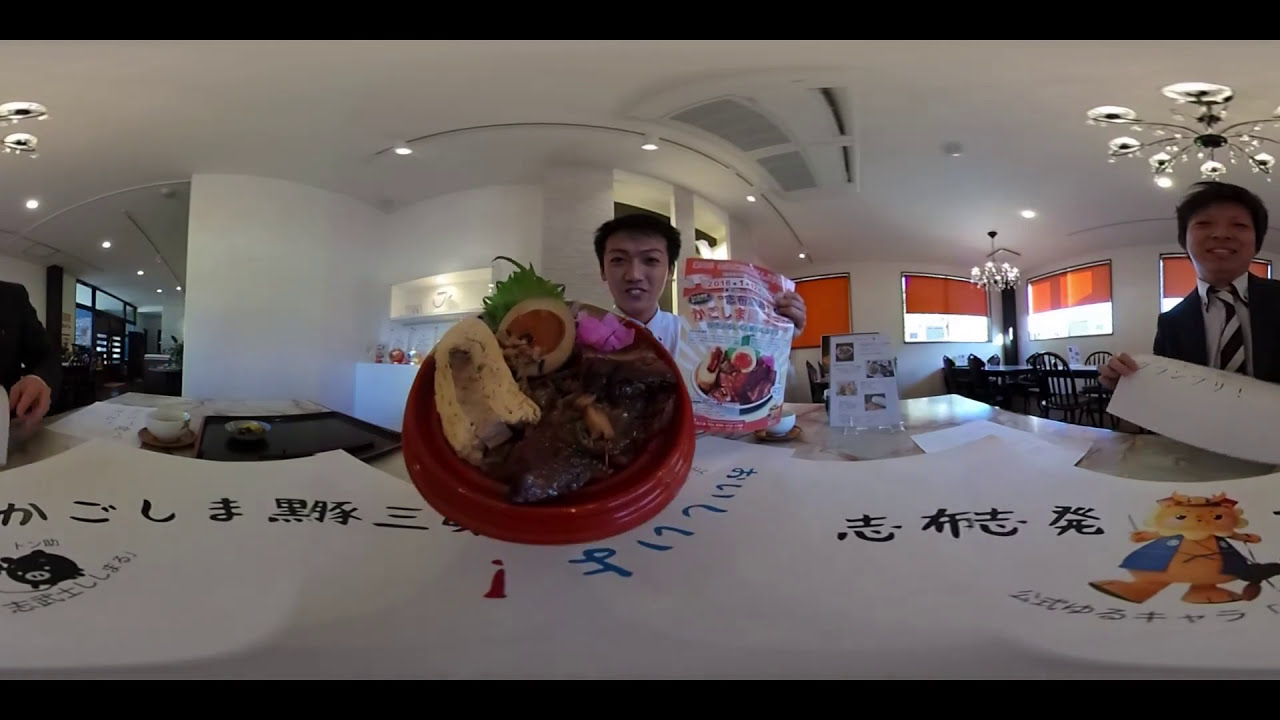The photo captures an indoor scene in what appears to be a hotel restaurant in Asia, discernible by the presence of oriental writing and a distinctly Asian plate of food. The room features white walls and ceilings, accentuated by white vents and chandelier-like silver lights. Orange blinds partially cover the windows, with some open and some closed, allowing a glimpse of the outside.

Three men are visible in the image. The leftmost man, whose face is partially cut off, wears a black suit and is picking up what looks like a white Chinese food box. Next to him, a white cup rests on a brown coaster beside a black tray with what seems to be a dish containing green and purple elements. The central figure, dressed in a white button-down shirt, holds a red plate piled with meats, rice, and possibly an egg in his right hand, and a plastic package depicting a similar meal in his left hand. The man on the right, clad in a dark suit with a black and white tie, holds a partially visible sign adorned with Japanese text, aligned with other Japanese text and characters on papers spread across the black and white table. These papers feature a blend of black, red, and blue text and illustrations, including an orange lion in a blue coat and a black and white pig.

The overall ambiance suggests an elegant dining setting, intensified by the fancy lighting and meticulously arranged table setting, underscored by the presence of various food items and detailed textual elements, solidifying the impression of an upscale Asian restaurant.